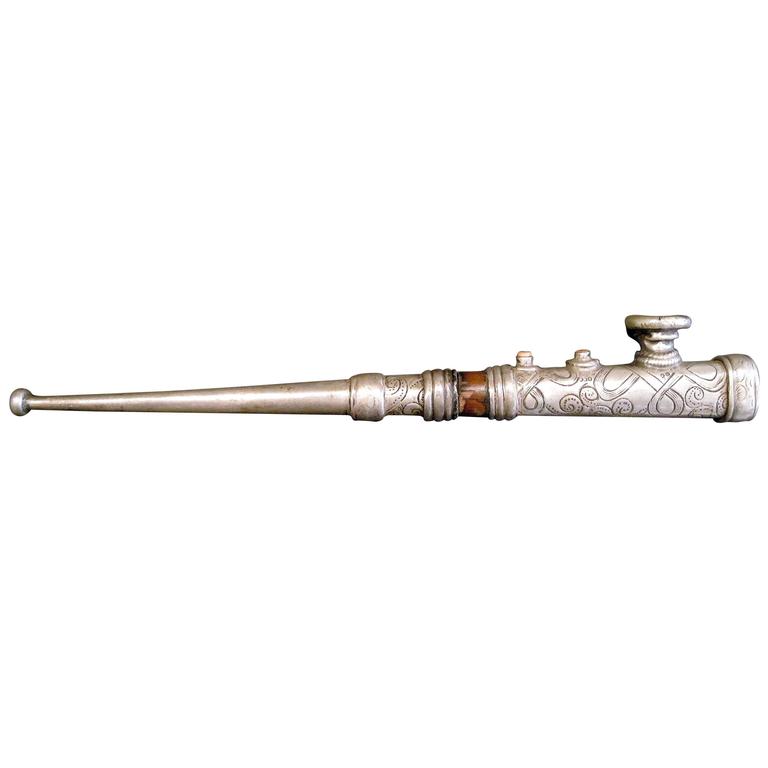The image depicts a cylindrical object that gradually enlarges from left to right, resembling the shape of a baseball bat. Positioned against a pure white background with professional lighting that minimizes reflections, the object's left side features a small knob, accentuating its thinner end. As it progresses to the right, the object thickens until it culminates in a wider section. Notable engravings adorn the surface, with ribbon-like patterns and wavy, snake-like lines accentuating its form. Midway along the object, a dark, shiny reddish-brown ring adds a striking artistic touch, possibly indicating a connection or decorative element. The top part of the object includes an area that appears designed for insertion, such as a compartment for tobacco, suggesting a possible functional aspect. The material is ambiguous, but it may be a painted wooden surface or even an animal tusk, contributing to its overall ancient and mysterious aura.